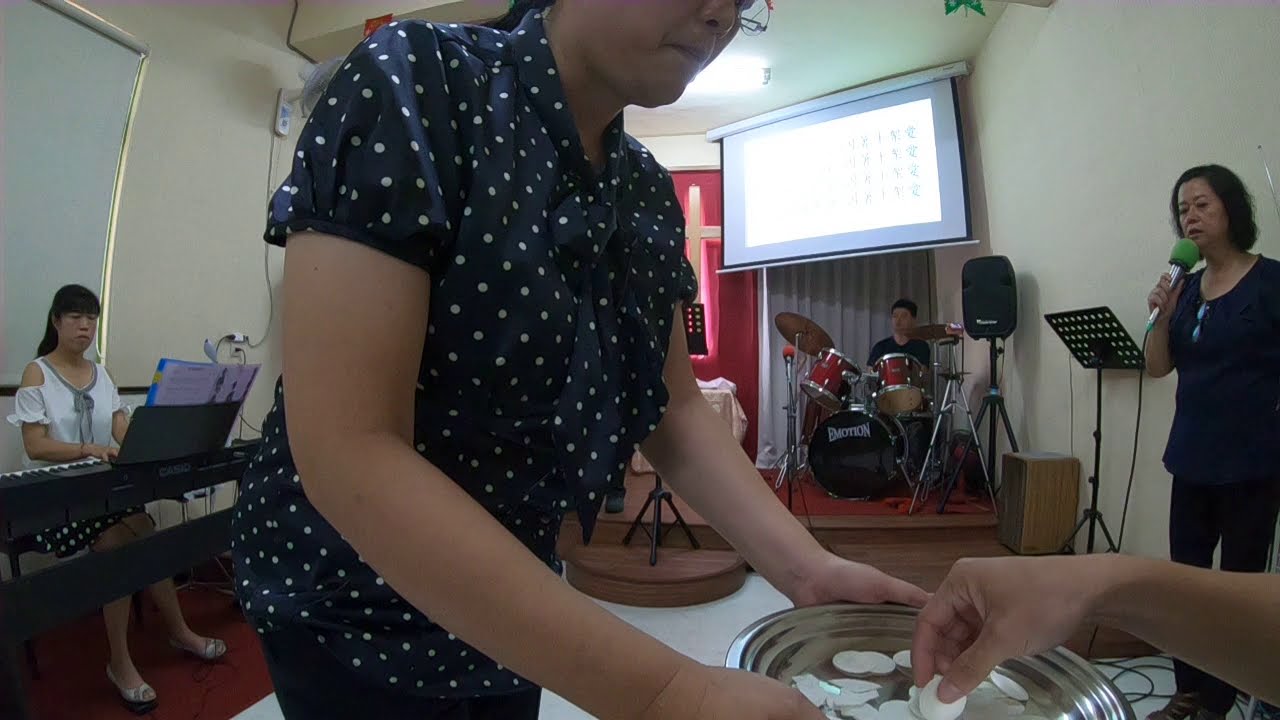In this horizontally-aligned rectangular image, we see a group of people engaged in various activities within a room that appears to be a church, characterized by a red curtain and a cross in the background. On the right side, a woman with short black hair and olive-colored skin is speaking or singing into a silver microphone with a green tip, while standing against a white wall. In the middle foreground, a woman in a navy blue and white polka-dot blouse, wearing glasses, is holding a tray with round white objects that resemble small chips or cardboard pieces. A hand from the lower right-hand corner is sticking these pieces onto the tray. To the left, another woman, dressed in a white cold-shoulder top and sitting at a keyboard, is looking at music sheets with a white wall and whiteboard behind her. In the background, partially obscured by a projector screen, a man in a black shirt is seated at, and possibly playing, a drum set. All of the individuals appear to be of Asian descent.